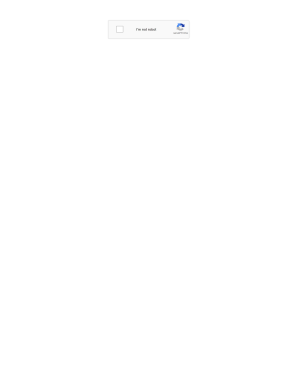In this image, towards the top, there is a prominent "I'm not a robot" CAPTCHA icon. It consists of a small gray rectangle. Inside the rectangle, on the left, there's a white checkbox. In the center, barely legible but recognizable, the text reads "I'm not a robot." On the right side of the rectangle, the brand name "CAPTCHA" is displayed, completing the image. The entire composition is simple yet functional, indicating a common online verification element used to distinguish human users from automated bots.